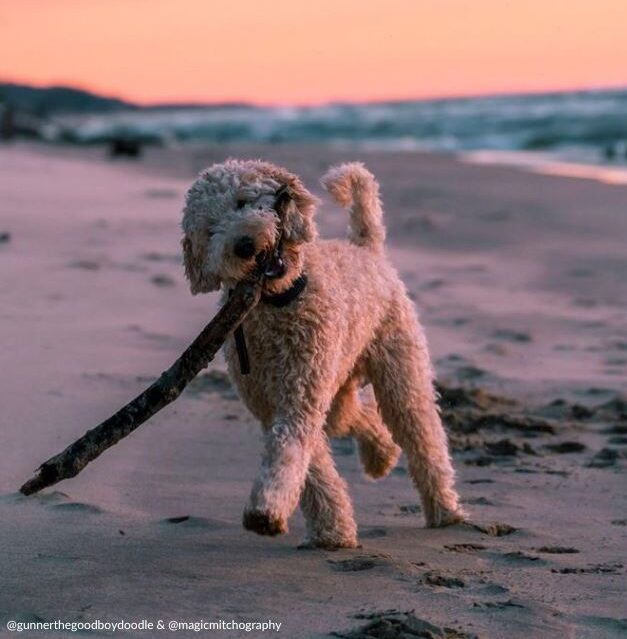A beautifully rendered professional photograph captures a playful poodle mix, likely a Labradoodle or Goldendoodle, with a velvety, whitish coat tinged pinkish-red by the sunset. The dog confidently races along a sandy beach, a large piece of driftwood clutched in its mouth and dragging to the sand below due to its sheer size. Its head is cocked to the side as it navigates with the stick, leaving a trail of footprints and paw prints behind in the brown sand. The ocean stretches out in the backdrop, merging with the darkening sky, painted in hues of pink and red by the setting sun. In the bottom left corner of the image, social media handles "@GunnertheGoodBoyDoodle" and "@MagicMitchography" are subtly inscribed, lending the scene a personal touch.